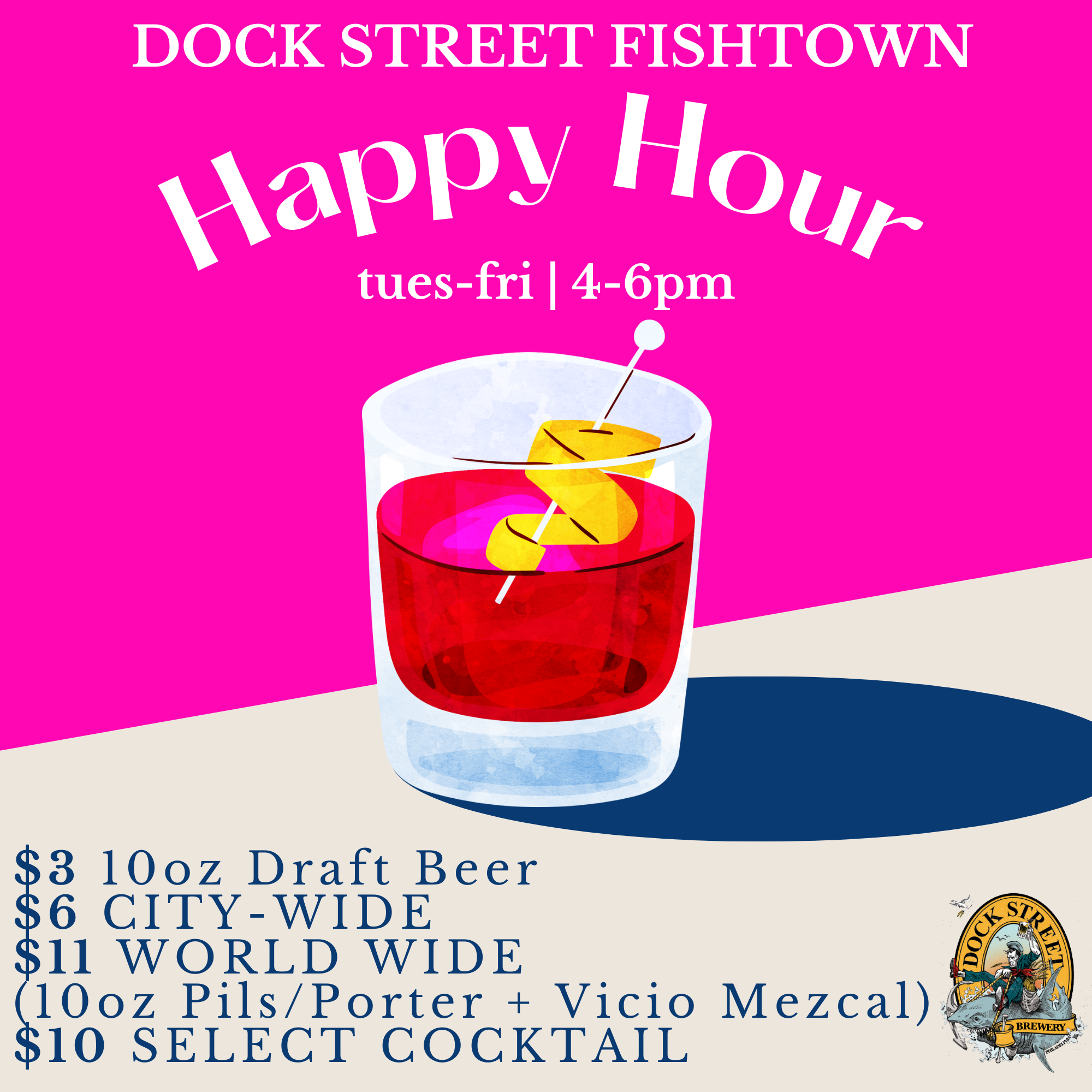This vibrant poster advertises Dock Street Fishtown's happy hour, juxtaposing a neon pink top half with an off-white bottom half. Dominating the center is a whimsical hand-painted illustration of a cocktail in a standard glass filled with a red liquid, garnished with an orange peel elegantly wrapped around a toothpick. The glass casts a shadow to the right, rendered in a blue hue. 

At the top of the poster, in striking white letters, it reads: "Dock Street Fishtown Happy Hour, Tuesday through Friday, 4 to 6 p.m." Towards the bottom left, a blue menu details the special prices: $3 for a 10-ounce draft beer, $6 for Citywide, $11 for Worldwide (10-ounce pilsner/porter plus Vickio Mezcal), and $10 for select cocktails. Finishing the design, the bottom right corner features a tiny, intricate logo of Dock Street Brewery, depicting a person riding what might be a dolphin, within a yellow oval frame, accentuating the overall playful yet sophisticated theme of the advertisement.